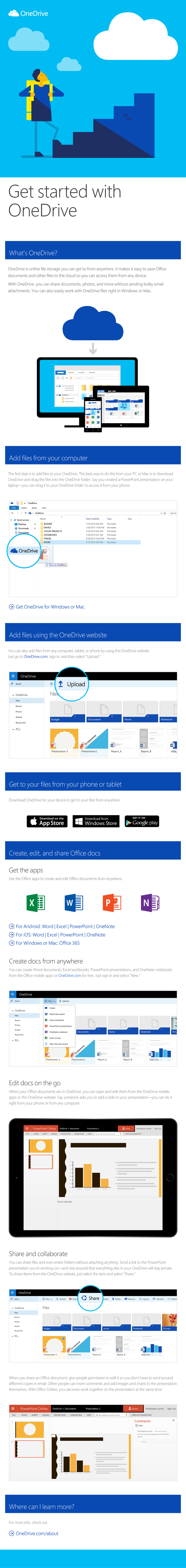Here's a cleaned-up and detailed caption for the described image:

---

The image depicts a low-quality, vertically compressed, and blurry screenshot of a generic website template. The template appears as a single cohesive design that presents an array of visual elements, though they are not clearly readable.

At the top, there is a blurry text that appears to read "Get Started with One Drive" set against a background showing a man with a backpack standing at the base of a staircase. The background has a blue sky with white clouds.

Below this headline, a series of elements are aligned vertically. First, a blue bar encompasses the width of the template. Below it, there is an illustration of digital devices, including a monitor, a tablet or laptop, and a cell phone, all connected to a blue cloud icon above them. 

Further down, there are several bars and sections which include indecipherable charts and graphs, some of which are highlighted and circled in blue. The overall clarity is poor, making it impossible to read any specific content or data presentations.

Towards the bottom of the image, there are several blue bars with black fields underneath that seem to be placeholders for icons corresponding to the Apple App Store and Google Play Store. There is another unidentified icon present as well.

The very last section features what seems to be a collection of Microsoft Office logos, including a green one typically associated with Excel, among others. The final elements include more charts and various data representations, which remain unreadable due to the image's low quality. The left side appears to show a cell phone with bar graphs, reinforcing the theme of data and digital connectivity.

The overall presentation is blurred and compressed, making it difficult to discern specific details and contributing to a chaotic and unclear visual experience.

---